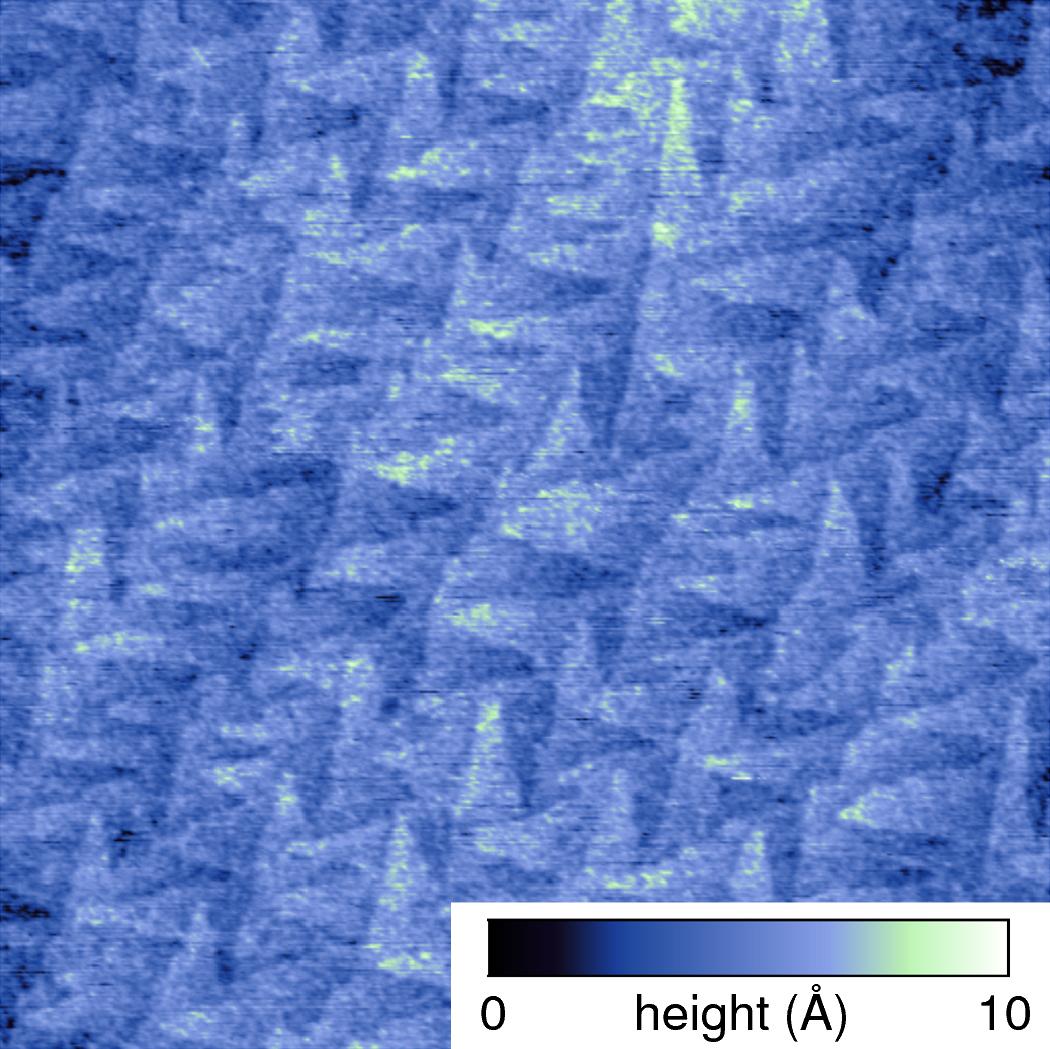The photo depicts an abstract image with varying shades of blue, periwinkle, black, white, and hints of light green. The dominant color is blue, which fades into different tones across the picture. The pattern consists of numerous superimposed triangles pointing in various directions, giving the image a layered, intricate texture. Positioned in the bottom right corner is a gradient scale, starting from dark blue at zero and transitioning through periwinkle and light green to white at ten, labeled "height (a)". The image suggests some form of scientific measurement or scanning device, capturing data through this abstract coloration. The middle and top sections are noticeably brighter compared to the dimmer left and top right edges, suggesting possible variances in the measured data, predominantly falling under the range of zero to five, with occasional peaks reaching up to ten.